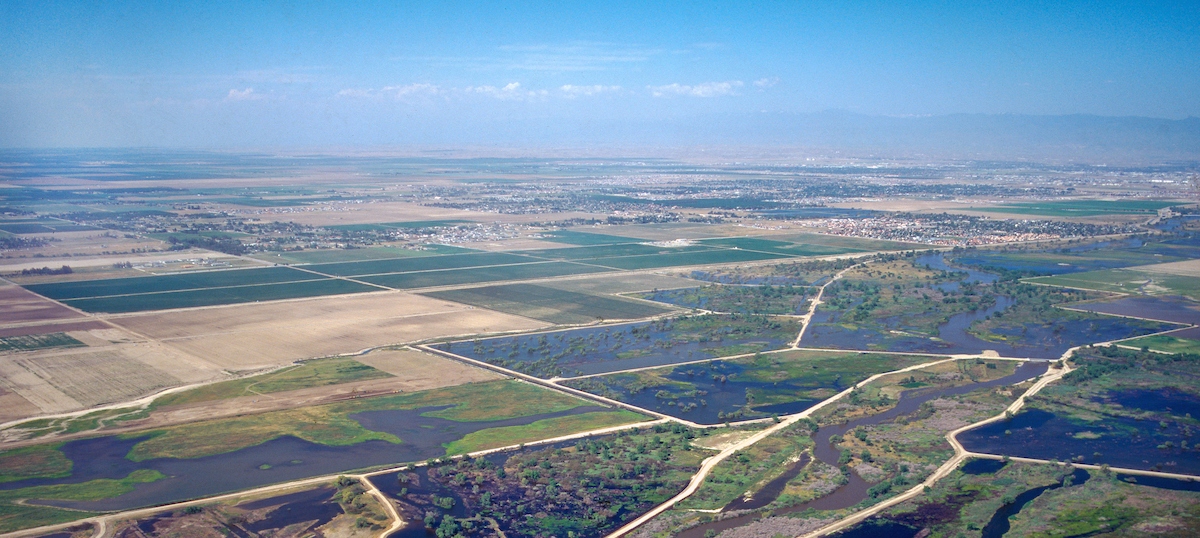Captured from an aerial vantage point, possibly from an airplane, this daytime image showcases a sprawling landscape below, characterized by a mix of water and land features. Dominating the scene are large bodies of water that intermingle with expanses of green and patches of bare earth, creating a vast, mosaic-like appearance that closely resembles a giant marshland. It gives an impression of an agricultural setting with parcels and patches of lush, green fields juxtaposed with bare, dirt areas. Notably, some parts seem inundated, with water visibly running through the grassy areas on the bottom left to right of the image, indicating possible flooding. Beyond this intricate patchwork, the horizon reveals a distant, blurred outline of a mountain or hilly terrain under a bright blue sky. Scattered clouds hover centrally in the image, adding to the picturesque vista. Far off in the distance, one can make out minute specks which suggest distant civilization, contrasting with the expansive, unbroken fields in the foreground. The serene sky complements the diverse and detailed landscape below, making for an evocative and detailed aerial scene.